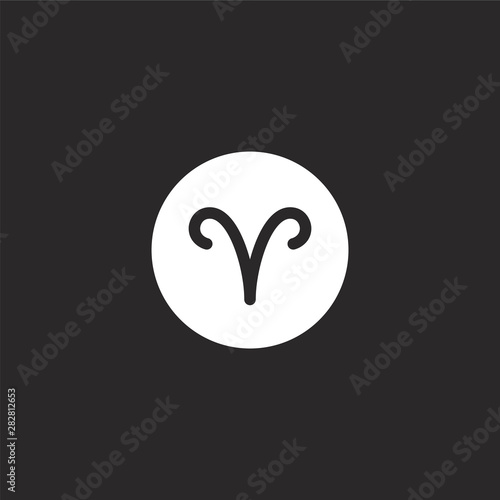This black and white graphical image presents a striking and minimalist design. Set within a matte dark gray square background, the focal point is a large white circle positioned centrally, occupying roughly a third of the image. Within this circle lies a stylized black 'V', notable for its thick, curved lines that evoke the shape of antlers or ram's horns. The design gives the impression of two candy canes placed together, curving upward and outward before bending inwards again.

Subtle but distinct, an Adobe Stock watermark in light gray diagonally traverses the background, repeating in a pattern. The font is faint yet readable, ensuring the branding does not detract from the main visual. Additionally, the bottom left corner of the image includes the Adobe Stock text in white, accompanied by the serial number 282812653, which can be used to locate this specific graphic in the Adobe Stock library. The overall style of the image leans heavily into clean, modern graphic design with a monochromatic palette.